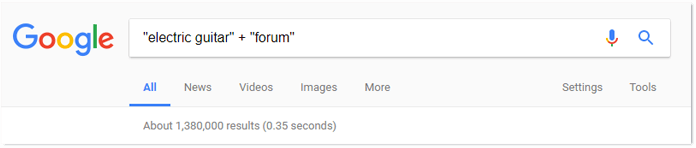This image captures a Google search results page with the following layout and elements: At the top left, the Google logo is prominently displayed, featuring a capital blue "G," followed by a lowercase red "o," yellow "o," blue "g," green "l," and red "e." Next to the logo is the familiar Google search box, a large rectangular area shaded in gray with a white search field inside it. The search field contains the text `"electric guitar" + "forum"` indicating the search query. To the right of the search box are icons for a microphone and a blue magnifying glass, representing voice search and the search button, respectively.

Below the search box, the search results page displays several navigation options. The words "All," "News," "Videos," "Images," and "More" are listed in a horizontal row; "All" is in blue with a blue underline, indicating the active tab, while the others are in gray. To the far right are additional options labeled "Settings" and "Tools" in gray. Directly beneath this menu row, a small white line appears.

Further down, the search results page indicates the number of results and the time taken to generate them: "About 1,380,000 results (0.35 seconds)."